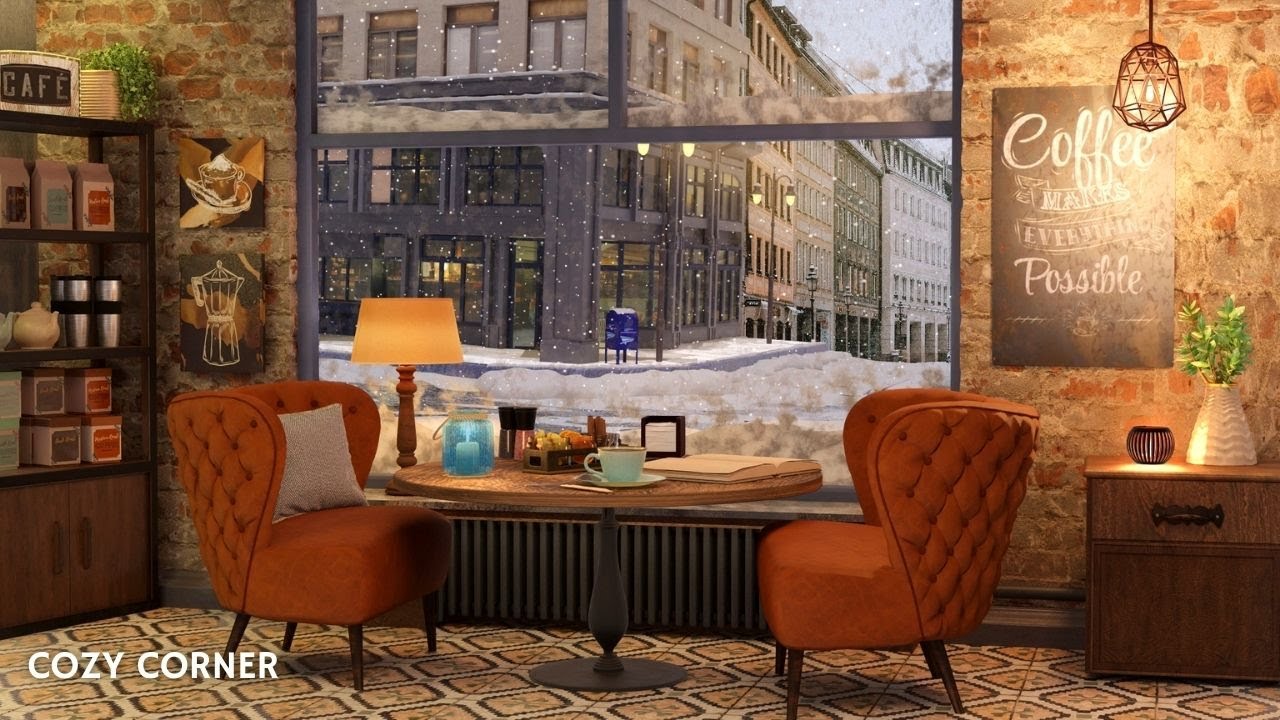In this highly realistic painting titled "Cozy Corner," the scene is meticulously detailed to evoke a sense of warmth and comfort. At the forefront, two rust-colored padded chairs are positioned at a round table, which is adorned with an open book, a blue coffee cup, a blue cylindrical candle, and a tray of condiments. A heat register is discreetly tucked beneath a large picture window that offers a clear view of the snowy exterior. Through the window, a blue post office mailbox stands against a backdrop of tall buildings, possibly part of a shopping center, all blanketed in snow with more flakes falling gently from the sky.

Inside, the ambiance is further enhanced by a stone wall, upon which a plaque with the phrase "Coffee Makes Everything Possible" is mounted. Below the plaque, a table holds a vase filled with lush greenery. Overhead, a pendant light casts soft illumination across this cozy setting. The opposite wall features a bookshelf that displays silver coffee cups, a sign reading "Cafe," and various pieces of decorative artwork, harmoniously integrated into the stone wall's texture.